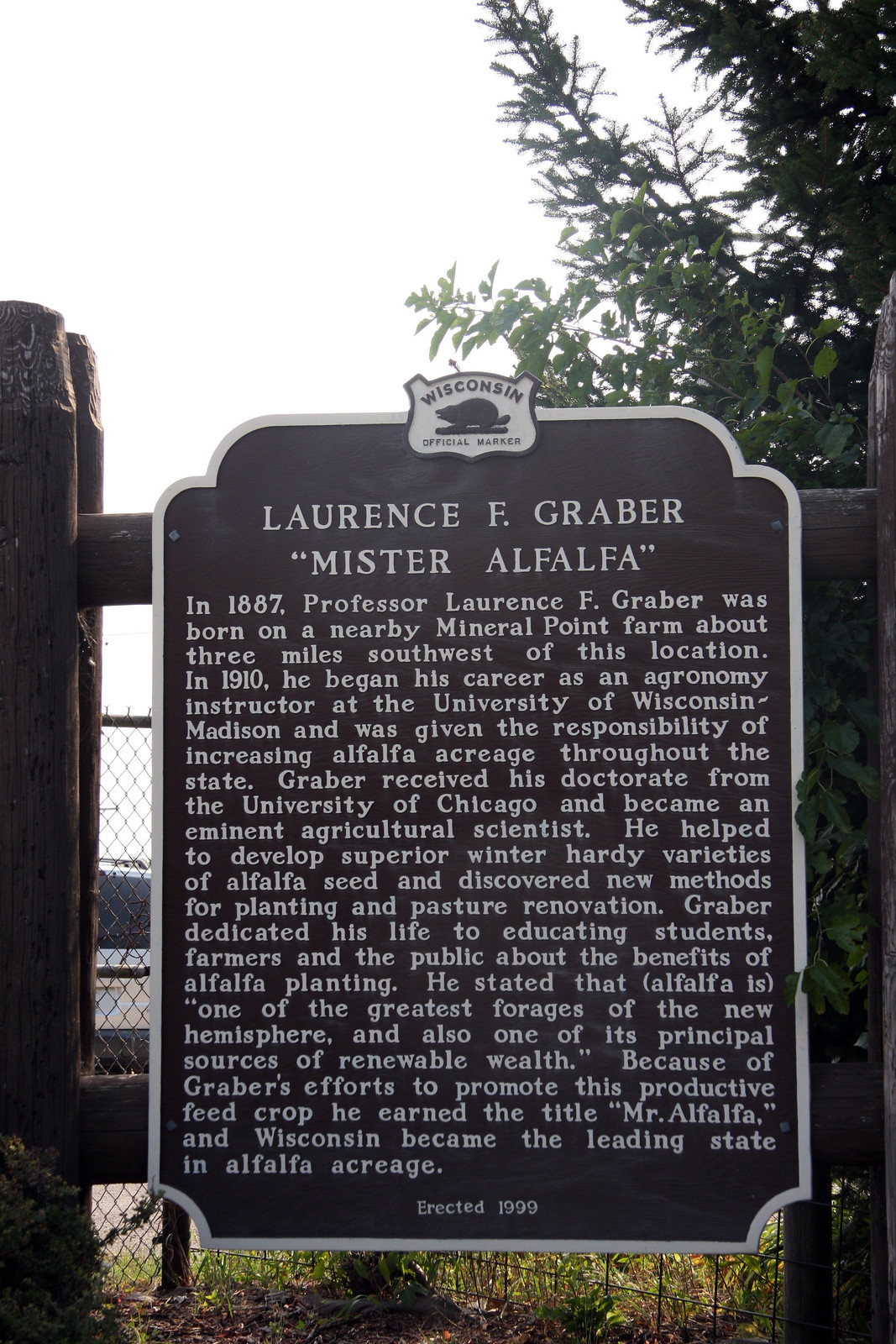This image depicts a historical marker in Wisconsin, prominently featuring a dark brown or black placard bordered in white. The marker commemorates Professor Lawrence F. Graber, fondly known as "Mr. Alfalfa," detailing his major contributions to agronomy. Born in 1887 near this location, Graber became a pivotal figure in promoting alfalfa cultivation, earning a doctorate from the University of Chicago. He later served as an agronomy instructor at the University of Wisconsin-Madison, where he developed winter-hardy alfalfa varieties and innovative planting methods. Due to his efforts, Wisconsin led the nation in alfalfa acreage. The marker, established in 1999, is supported by thick wooden posts and situated on a brown fence, with an evergreen tree visible in the background. Partial views of a car and what appears to be a parking lot can be seen beyond the fence, and the sky is a featureless white, typical of a bright day. On the top of the placard, the Wisconsin state emblem is displayed, affirming its historical significance.